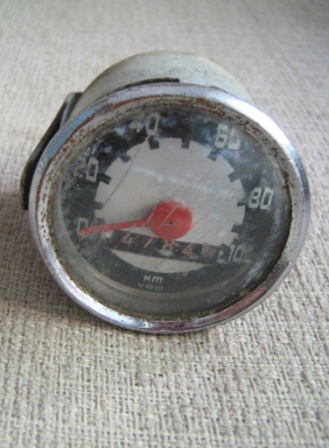This image captures a small, round speedometer placed on a piece of white cloth with a woven pattern. The speedometer, likely originating from a motorbike or moped, features a metal rim with a silver finish that's noticeably worn, revealing patches of rusty, bronze-colored metal beneath. The dial on the speedometer displays kilometers per hour (km/h) ranging from 0 to 100. The face of the speedometer is a striking contrast of black and white, with a red needle indicating the speed. Below the needle, a smaller mileage dial is visible. The overall condition of the speedometer suggests it's seen considerable use, adding a vintage aesthetic to the scene. The device measures approximately two to three inches in diameter.